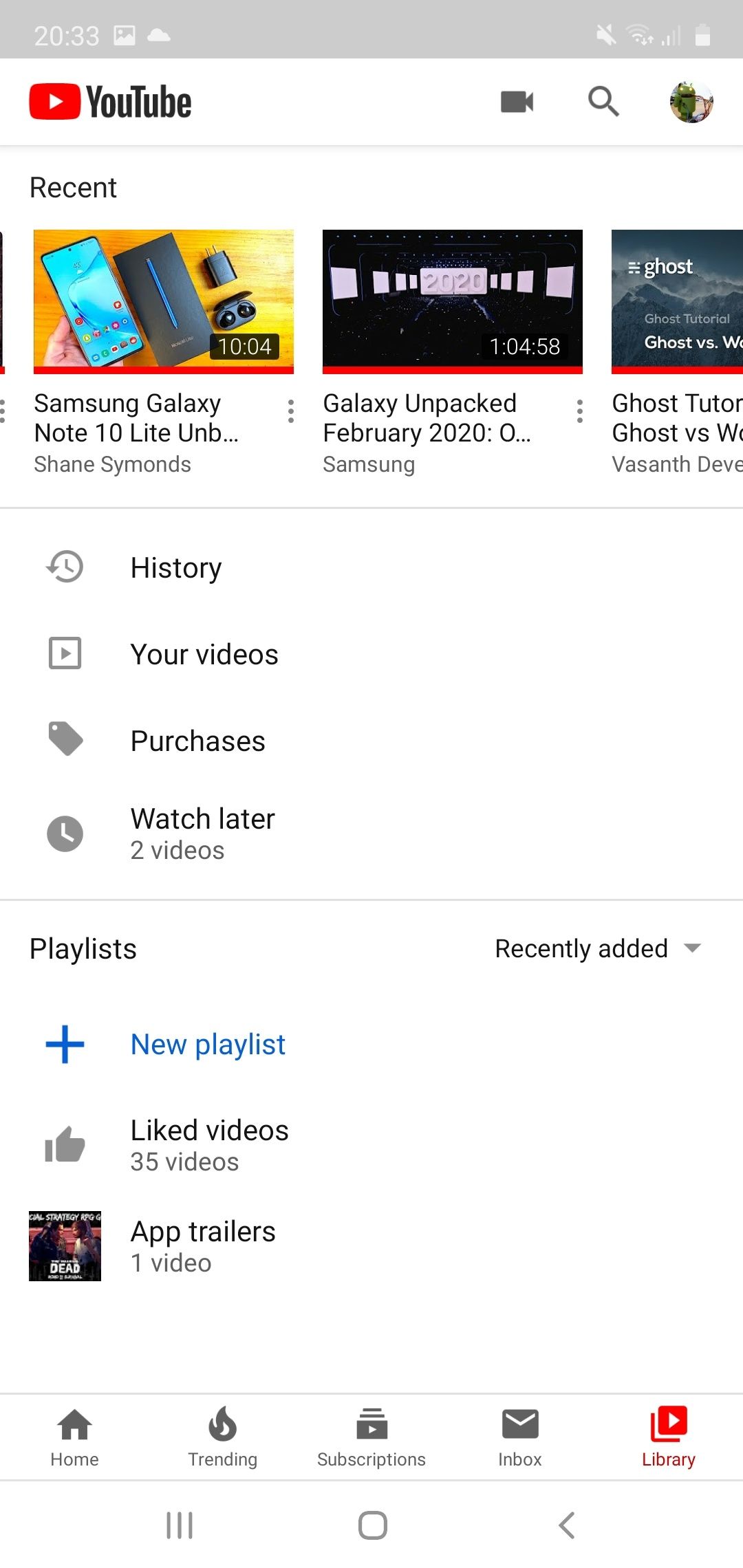The image portrays an Android phone screen displaying the YouTube app interface. At the top, a gray status bar shows the time as 20:33 in white. The ringer is muted, indicated by a line through its symbol. The device has one bar lit on the Wi-Fi signal, two bars on the network signal, and a person icon likely denoting a user profile or notifications.

Below the status bar, the YouTube app's header displays 'YouTube' on the top left, accompanied by a camera icon, a search icon, and a user's profile icon on the top right, though the profile picture is not clearly visible.

In the 'Recent Videos' section, two videos are prominently displayed. The first video is titled "Samsung Galaxy Note 10 LE Unboxed" by Shane Simons, lasting 10 minutes and 4 seconds. The thumbnail features images of the front and back of an Android phone. The second video is "Galaxy Unpacked February 2020" by Samsung, with a duration of 1 hour, 4 minutes, and 58 seconds, showing a thumbnail focused on the device screens. Both videos have fully red progress bars, indicating they have been completely watched. A partially visible video titled "Ghost Tutor, Ghost vs. [unreadable text] by Vasneth Devon" is also mentioned.

Further down, the screen lists various user options such as 'History,' 'Your Videos,' 'Purchases,' 'Watch Later' (noting two checked-out videos), and 'Playlists.' The 'Playlists' section features a dropdown menu labeled 'Recently Added,' options to create a 'New Playlist,' and a playlist titled 'Liked Videos' containing 35 videos marked with a plus symbol for easy access.

Additionally, there is an 'App Trailers' playlist mentioned, which comprises one video, but the details remain unclear. The bottom navigation bar of the YouTube app includes quick links to 'Home,' 'Trending,' 'Subscriptions,' 'Inbox,' and 'Library.'

Finally, at the bottom-most part of the screen, typical Android navigation buttons are visible: three horizontal bars for the menu, a square for recent apps, and an arrow for the back function.